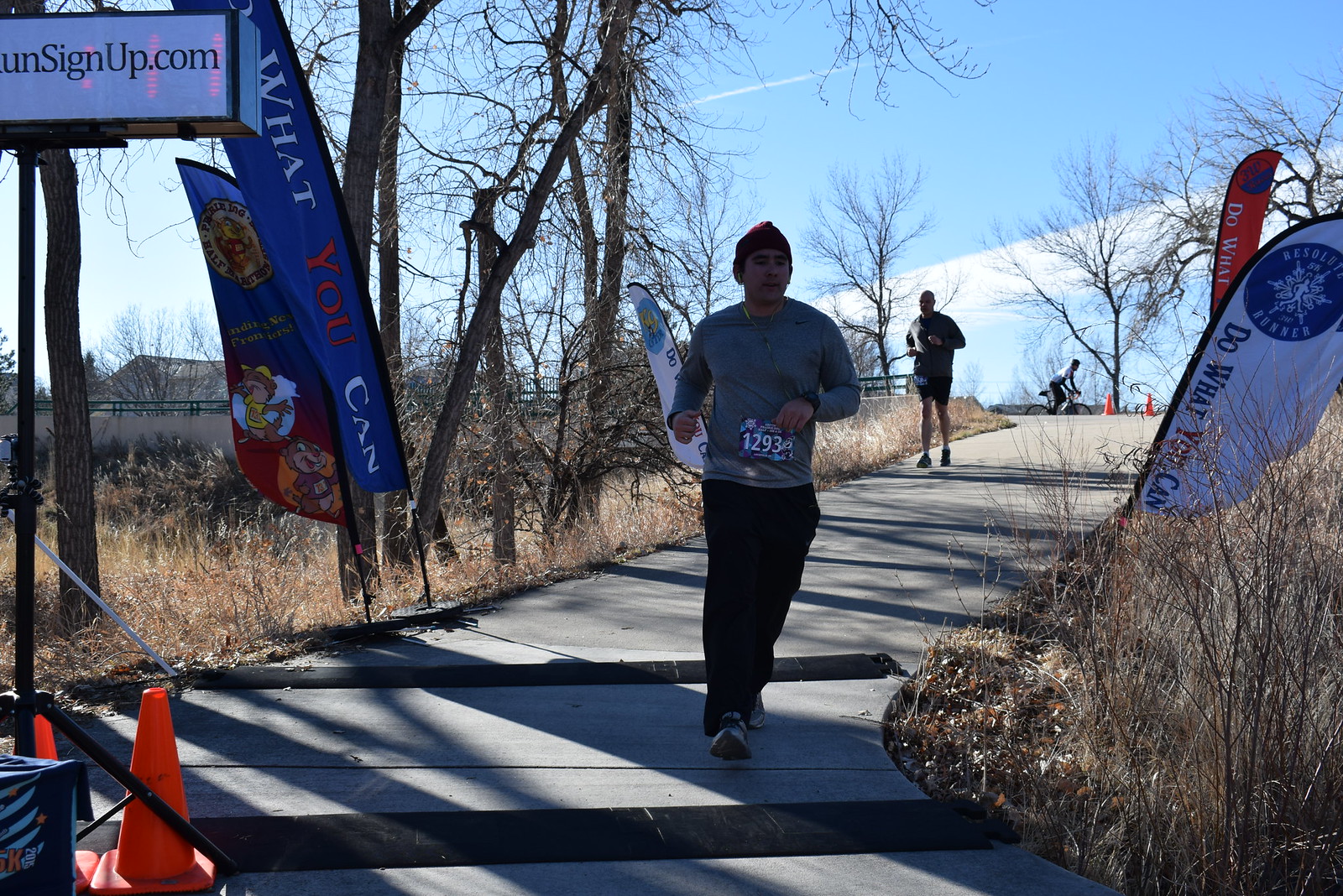The image depicts a road race on a cold day, evidenced by the runners' attire and the leafless trees surrounding the path. In the foreground, a runner wearing a blue jersey, black running pants, a cap, and a tag labeled "1293" is crossing what appears to be the finish line, stepping over black tape that likely houses sensors. This runner sports Nike gear, reflecting the chilly weather. Behind him, a second runner in jogging shorts and a long-sleeve jersey is also visible, though their tag is unreadable. Further in the background, there is a cyclist unassociated with the race. The race path is clearly marked with orange cones and features various banners on either side, including those with slogans like "signup.com" and "do what you can" in red, white, and blue. The scene is set during the daytime amidst barren trees and dormant grass, contributing to the overall wintry atmosphere.